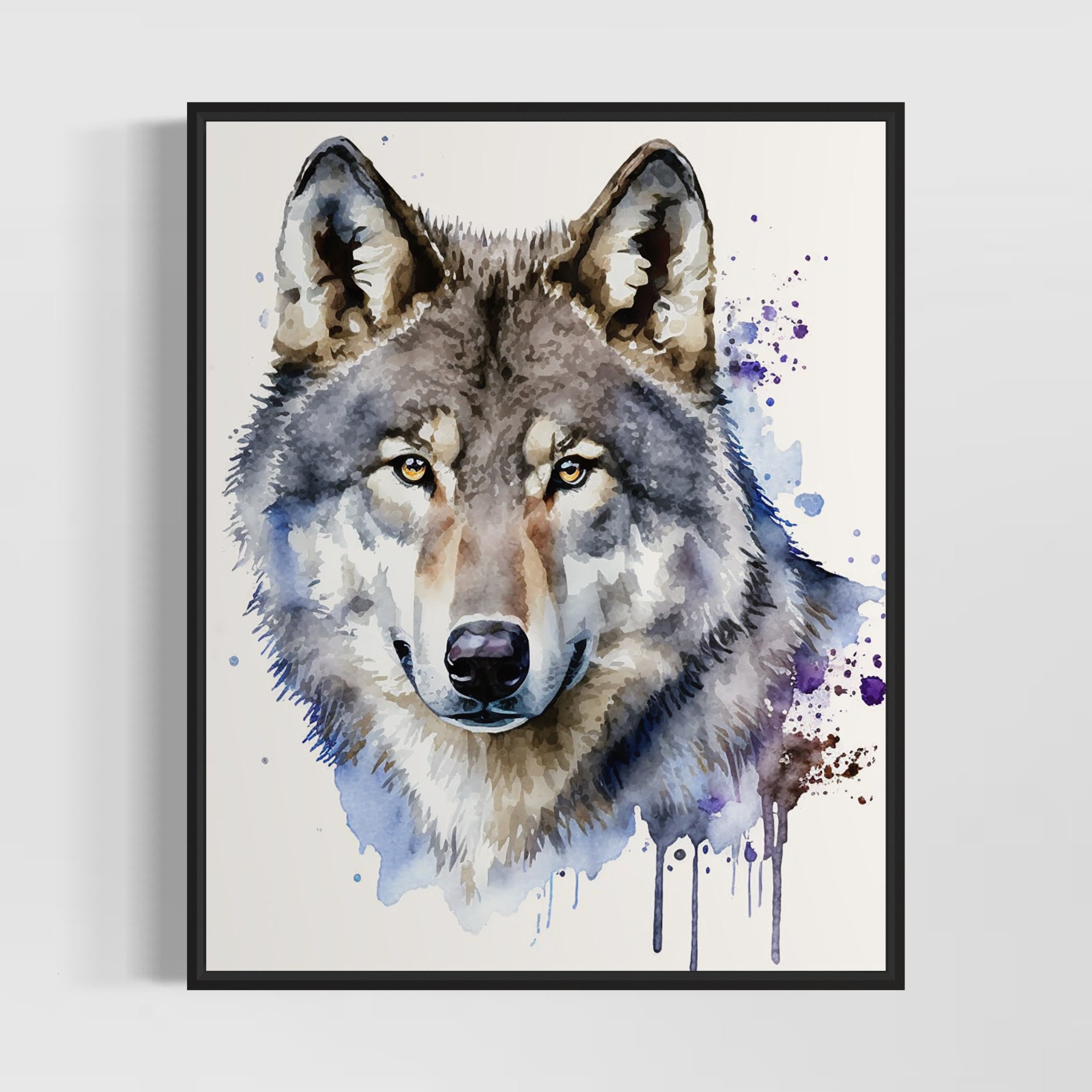This image features an exquisite watercolor painting of a wolf's face, encased in a thin black frame and mounted against an off-white, eggshell-colored wall. The wolf, depicted in a close-up, frontal view, commands attention with its striking amber eyes, black nose, and black mouth. Its fur is rendered with remarkable detail, showcasing a spectrum of grays, browns, and whites, with additional accents of blue and purple. The ears are pointed straight up and exhibit darker interiors. Notably, various shades of purple and blue paint create artful drips and splatters around and beneath the wolf's head, emphasizing the watercolor medium. The intricate interplay of light and dark grays gives the wolf's fur a dynamic, lifelike texture. This composition captures both the majesty and the delicate artistry of the animal, making it a stunning focal point.